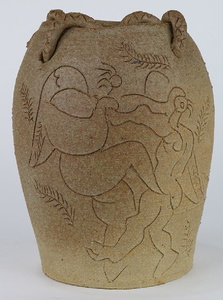This color photograph showcases a meticulously crafted piece of light brown pottery. The vessel features a gracefully curved top and a flat base, giving it a sturdy, yet elegant structure. Adorning the top rim is a decorative rope-like design, threaded through small holes, adding a touch of artisanal charm. The surface of the pottery is skillfully etched with intricate designs, including a detailed line drawing of two figures that appear to be dancing, accompanied by etchings of delicate branches. The pottery is captured on a pristine white surface with a seamless white background, ensuring all attention is drawn to its exquisite craftsmanship.